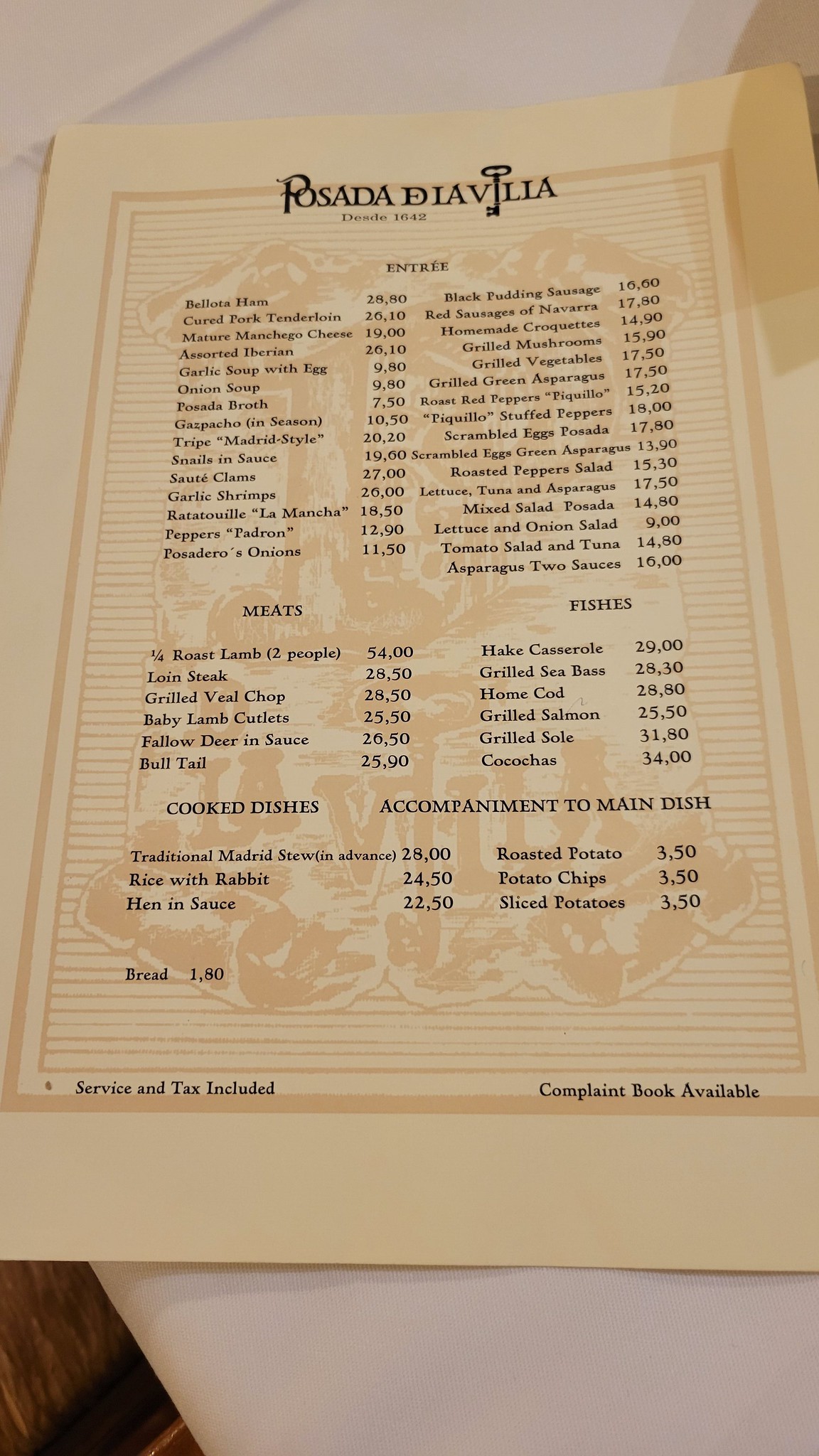A detailed photograph captures a restaurant menu placed on what appears to be a white tablecloth, with a hint of a brown wooden surface visible in the lower left-hand corner. The menu itself is of a delicate, very pale gold or peachy hue. At the top of the menu, the bold title reads "POSADA DIAV", followed by the letters "LIA" which are separated by a design element resembling a key. Beneath this title, there is some smaller writing that is not legible. The background features light beige horizontal lines and some form of an image that is too faint to be identified, overlaid by the menu's text.

The menu is divided into several sections, each denoting a different category of dishes. Under the "Entrees" section, some highlighted items include ham priced at $28, garlic soup with egg, onion soup, cured pork tenderloin, garlic shrimp, black pudding sausage at $15.50, and red sausages, with a total of at least 20 entree options.

On the left-hand column under the "Meats" section, options like roast lamb for two at $54 and loin steak at $28.50 are listed, continuing down to veal chops and other selections. In the "Fishes" section on the right, dishes such as hake casserole at $29 are mentioned along with several other fish options.

Below these sections, the left-hand side features "Cooked Dishes" while the right-hand side lists "Accompaniment to Main Dish" with items such as roasted potato, potato chips, and sliced potatoes, each priced at $3.50. Further down, "Bread" is available for $1.80. At the bottom of the menu, a note states "Service and tax included, complaint book available."